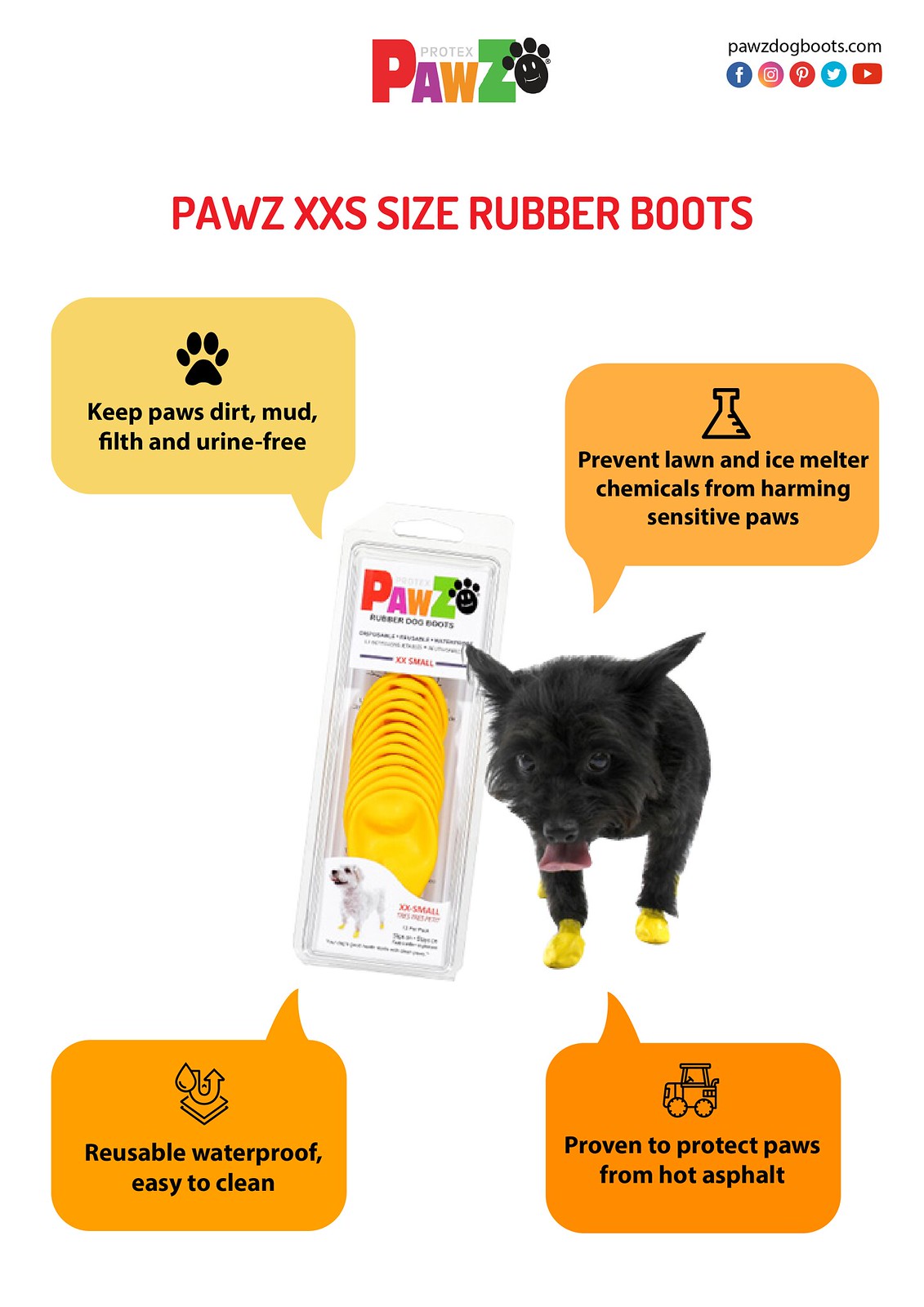This advertisement prominently features an array of elements to illustrate and market the "PAWS XX-small Size Rubber Boots" for dogs. At the top, the word "Protex" is followed by "PAWS" in colorful letters beside an image of a paw with a smiley face on the footpad. Adjacent to this, in smaller black letters, the URL "PAWSdogboots.com" is present, along with icons for Facebook, Instagram, Pinterest, Twitter, and YouTube. Central to the image is a clamshell plastic container filled with small yellow boots, labeled "PAWS," and beside it, a black dog is depicted wearing the yellow boots with its tongue playfully sticking out. The upper left section above the dog and boots prominently features the caption "Keep PAWS dirt, mud, filth, and urine free," while the lower right section states, "Prevent lawn and ice melter chemicals from harming sensitive PAWS." At the very bottom, two notable orange rectangles highlight the features: "Reusable, waterproof, easy to clean" on the left, and "Proven to protect PAWS from hot asphalt" on the right, all underscoring the practicality and protective qualities of these dog boots.